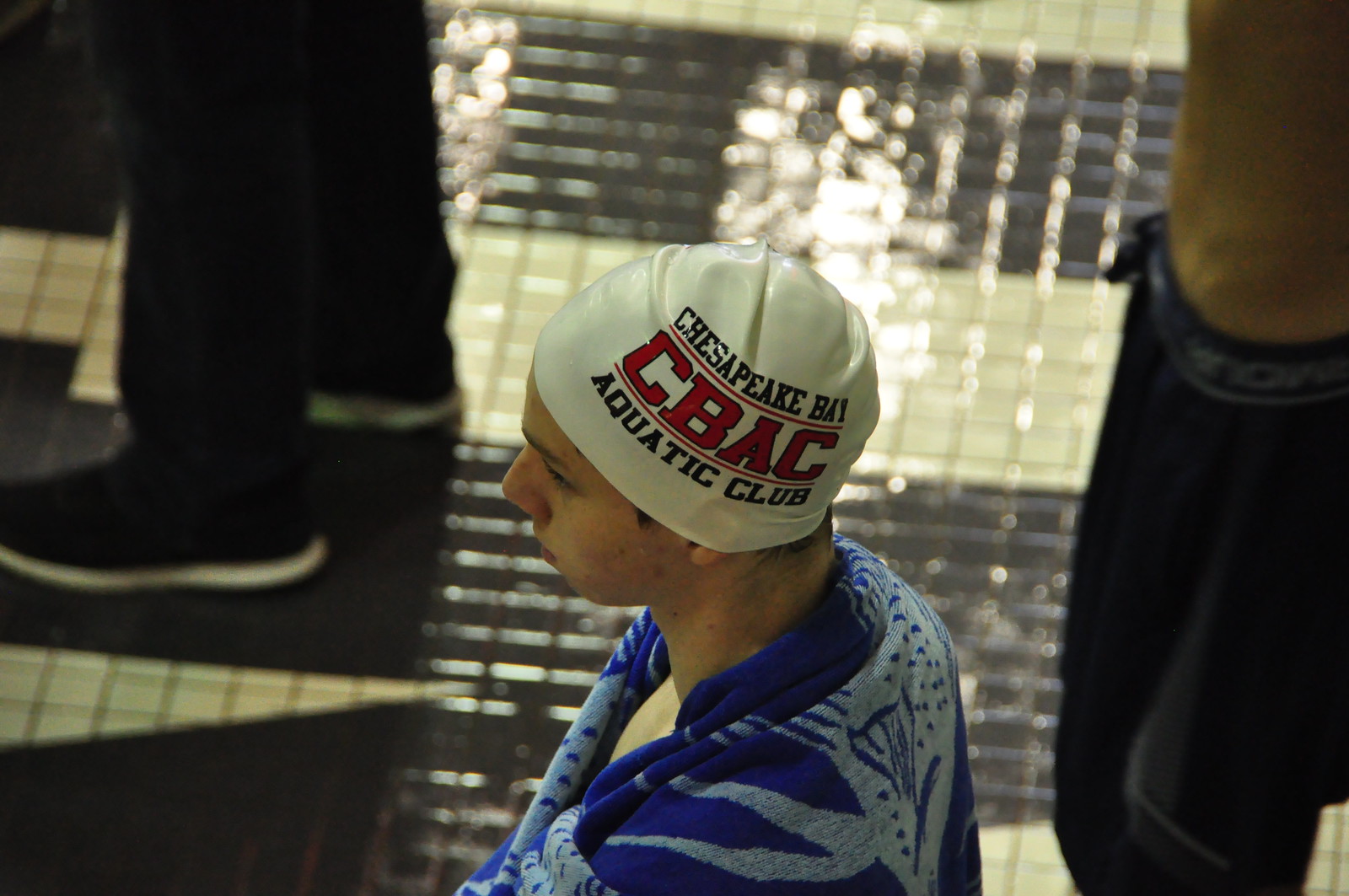The image depicts an indoor pool setting captured from an elevated angle. At the center of the frame is a swimmer, wrapped in a blue and light blue graphic towel, with a white swim cap that prominently features "Chesapeake Bay CBAC Aquatic Club" in large red and black letters. Though difficult to distinguish the gender, the swimmer appears to be a young male. He stands on a wet, black-and-white tiled floor, its shiny surface reflecting the indoor lighting. The swimmer's cap covers his ears and the towel drapes over his shoulders, suggesting he has recently exited the pool. Flanking him are partial figures: to the left, a person in dark pants and black shoes, visible only up to the knees; to the right, an arm clad in a dark sleeve and a torso in black shorts. This zoomed shot, likely taken from the stands during a swimming competition, focuses closely on the swimmer, emphasizing the detailed elements of his attire and the surrounding environment.